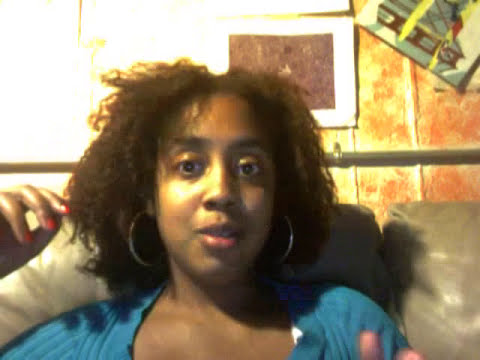In this image, we see a young African-American woman with shoulder-length, curly, dark brown hair. She's facing the camera with wide-open, dark eyes, and is wearing large gold hoop earrings and a blue blouse with a low-cut collar. Her right hand, adorned with red nail polish, is raised slightly towards her face. She is seated on a shiny gray leather couch, with a background that features a bright light source illuminating her from the upper left, causing a noticeable glare on her face and fingers. The wall behind her is primarily orangish with some parts appearing white, adorned with various posters and signs. The setting appears to be indoors, in a living room, giving the impression that this image might be from a live stream or a social media video, capturing her in the act of speaking.